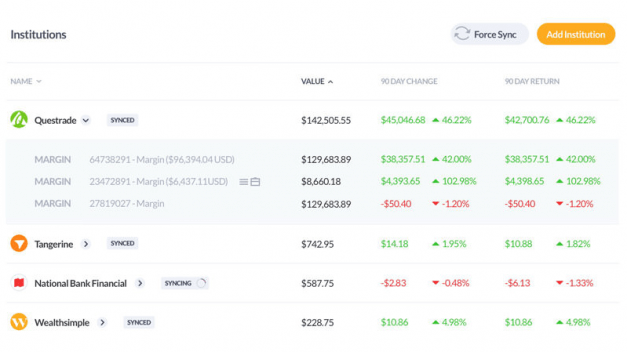The image is a horizontally rectangular screenshot from a financial application, displayed on a white background. At the very top left of the frame, the bold text "Institutions" is prominently featured. On the top right are two buttons labeled "Force Sync" and "Add Institution."

Below this header is a chart with four columns, titled (from left to right): "Name", "Value", "90 Day Change", and "90 Day Return." Under the "Name" column, there are four financial institutions listed: Quest Trade, Tangerine, National Bank Financial, and Wealth Simple.

All the corresponding financial figures for each institution are populated under the "Value," "90 Day Change," and "90 Day Return" columns. Additionally, Quest Trade has a dropdown menu that is expanded, revealing three individual listings beneath it, each with their own detailed numbers filled in the respective columns.

The overall layout is clean and organized, providing a clear summary of each institution's recent financial performance.